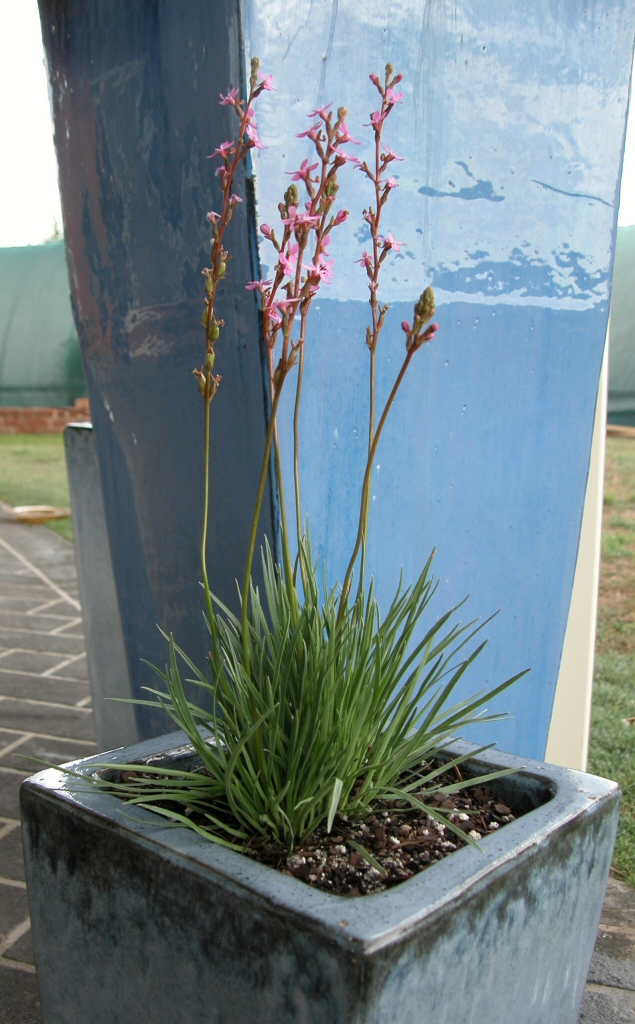The image features a large, gray ceramic planter situated outdoors on a brick-type walkway. The planter, which appears heavy and thick, stands about one and a half to two feet tall and has a shiny, hand-glazed finish that transitions from lighter at the bottom to a darker gray near the top, with the lip returning to a lighter shade. Inside the planter, a plant with green leaves is growing, accompanied by tall shoots that bear buds just beginning to open into tiny pink flowers. The base of the planter contains a mix of dirt and small white rocks. The planter leans slightly against a shiny post, likely a power or light pole. Also leaning against this post is a metal sheet that reflects the color of the sky and the sun. The background features grass and a green fence atop a brick wall.